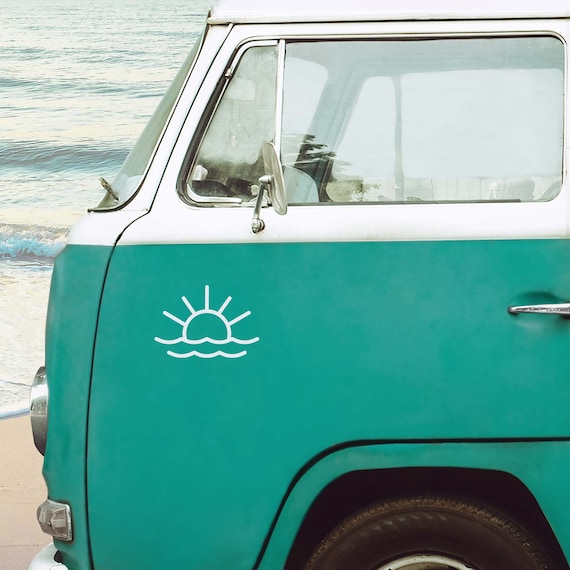This photograph showcases a front driver's side view of a classic VW bus, affectionately known as a VW van. The top half of the bus is painted white, while the bottom half sports a striking turquoise-teal color. Prominently displayed just beneath the driver's side mirror is a white, line-drawn sun with two wavy lines underneath, symbolizing ocean waves. The bus, parked on a sliver of sand at the edge of the beach, is positioned extremely close to the ocean. The background reveals gentle waves lapping against the shore, indicating a serene, slightly sunny day. The windows of the van are rolled up, reflecting the sunlight, and a single black tire is visible in the foreground.